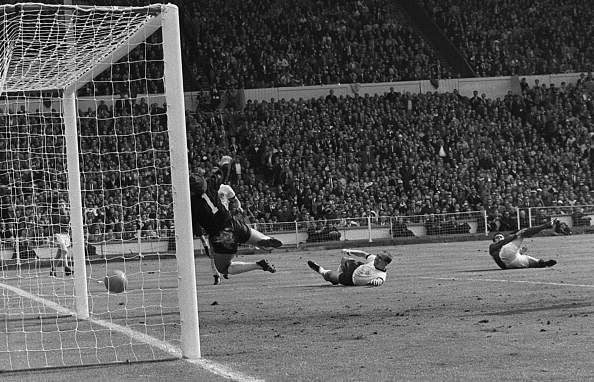The black-and-white image captures an intense moment during a soccer game in a packed, two-level stadium with thousands of spectators. The focus is on the field where five players are visible, with two lying on the ground near the goal post on the left side, possibly knocked over in the heat of the action. The goalie's dynamic attempt to block an incoming ball is the centerpiece of the scene; he's airborne, fully stretched out in his black jersey, reaching towards the left post. The four other players on the pitch wear white jerseys, with one seemingly responsible for the decisive kick. Notably, the soccer ball is devoid of the traditional hexagon and pentagon patterns, appearing uniformly white. The photograph's vintage style and black-and-white format suggest it may be from an earlier era, possibly the 1980s, adding a nostalgic championship game feel to the moment.